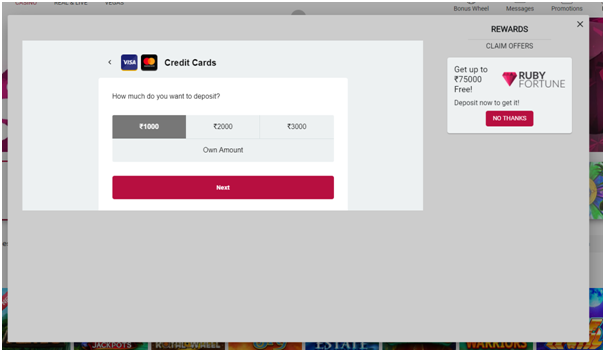A detailed descriptive caption for the image:

"This screenshot captures a website interface overlaid by a prominent grey pop-up window covering the majority of the screen. In the top-right corner of the pop-up, the word 'Rewards' is displayed alongside an 'X' button for closing the window. Directly below the 'Rewards' header, the text 'Claim Offers' appears with a small white input box beneath it. On the left side of the pop-up, a promotional message advertises, 'Get up to $75,000 free' with a foreign currency symbol. To the right of this message, the words 'Ruby Fortune' are shown next to a logo featuring a faceted ruby gemstone. Below this, the text 'Deposit Now to get it' encourages action, followed by a prominent red button labeled 'No Tax and No Tax.'

To the left of the red button, a lighter grey box outlines a section labeled 'Credit Cards,' displaying Visa and MasterCard logos at the top. This section prompts users to select an amount to deposit, presenting three options: $1,000, $2,000, and $3,000. An additional option labeled 'Own Amount' allows for custom entries. Completing this section is a red button labeled 'Next' situated at the bottom."